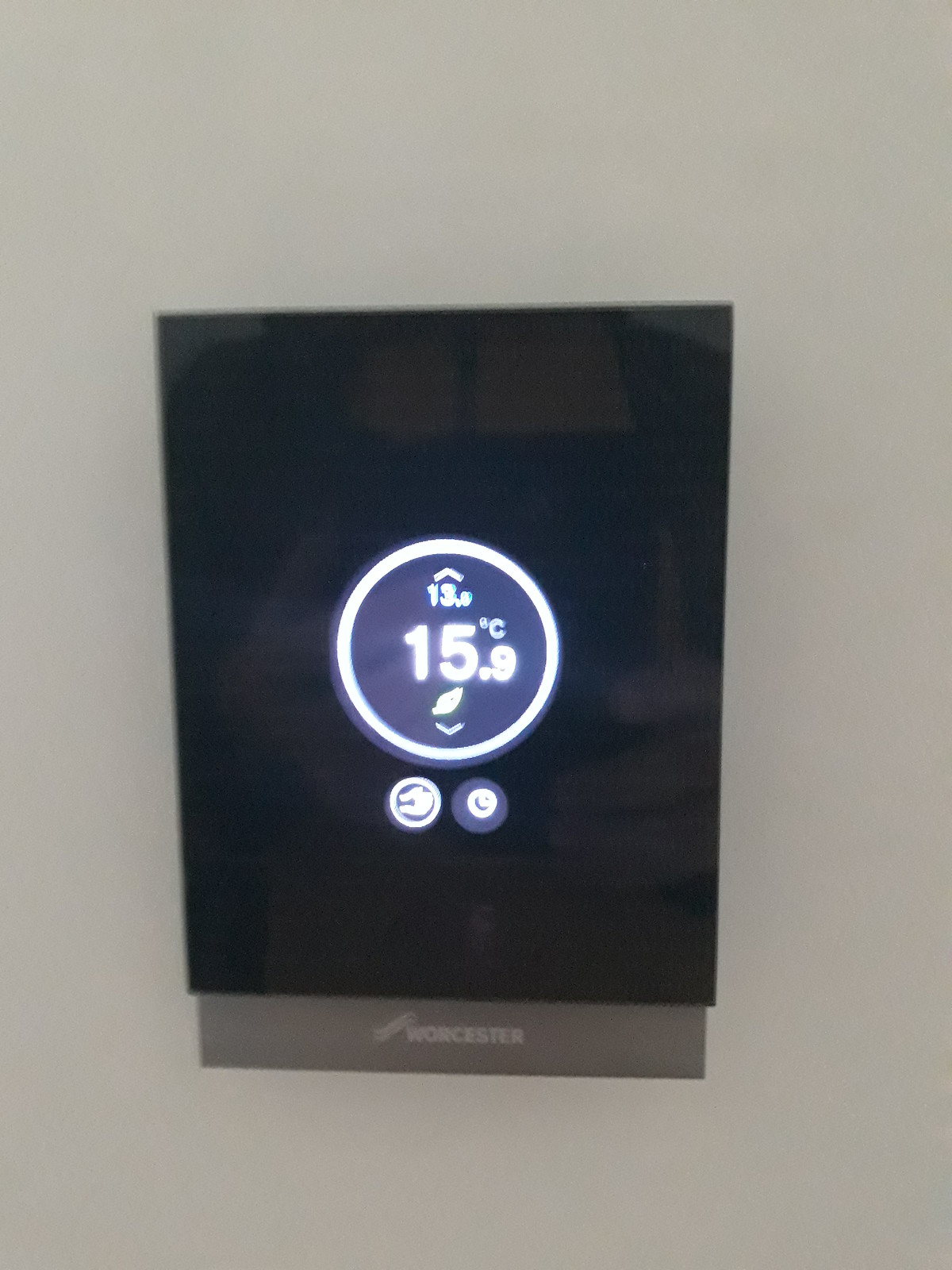The image displays a black square centered on a gray background, seemingly indicative of a temperature display. Inside this black square is a prominent white circle. Within the white circle, text readings in a vertical format are visible. At the top, partially hidden by an array, is "13.0," followed by "15.9" below it. The numerical reading intersects with the words "degrees centigrade" which are positioned near the top of the number "5."

Directly beneath this text, a white icon sits upon a downward-pointing caret symbol, also white. Flanking the lower edge of the white circle are two distinct buttons: a white-outlined circle with an icon at the center on the left, and on the right, a black icon featuring a white shape in its center.

Underneath the black square, a light gray banner stretches across the base, displaying an icon or logo alongside the word "WORCESTER" in bold, all capital letters. This word appears slightly shadowed, likely cast from the black square above, giving it a subtle three-dimensional effect against the gray backdrop.